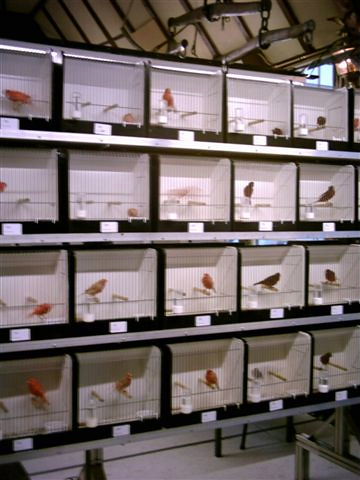This photograph, taken inside what appears to be an aviary display or pet store, shows a large collection of small bird cages arranged on shelves. Each cage measures approximately one cubic foot, with a black frame and white interior. The cages are set in a 4x5 grid, totaling 20 identical compartments. Each cage houses a solitary bird, with colors ranging from red and orange to various shades of brown. The cages, which have limited space, contain two wooden perches and a small bowl, likely for food or water. Above the shelves, the image captures a rustic wooden roof with beams and chains, adding to the rustic charm of the setting. Some cages also feature a water bottle and a small label, possibly for identification. Overall, the detailed scene suggests a carefully maintained display, albeit within tight and small confines for the birds.